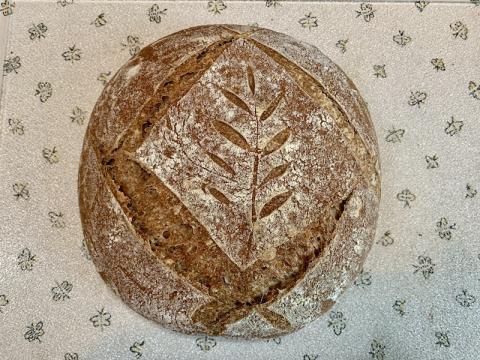The image depicts a rustic, circular loaf of hand-crafted bread, seated on an off-white tablecloth adorned with small brown butterfly prints. The bread is a relatively dark tan, almost light brown, with a dusting of flour creating white splotches. The most striking feature is the decorative pattern on top: a design resembling a branch with multiple leaves, artistically scored into the thick, crusty surface. The photograph captures a top-down view, emphasizing both the artisan details of the bread and the delicate butterfly motif of the tablecloth below.